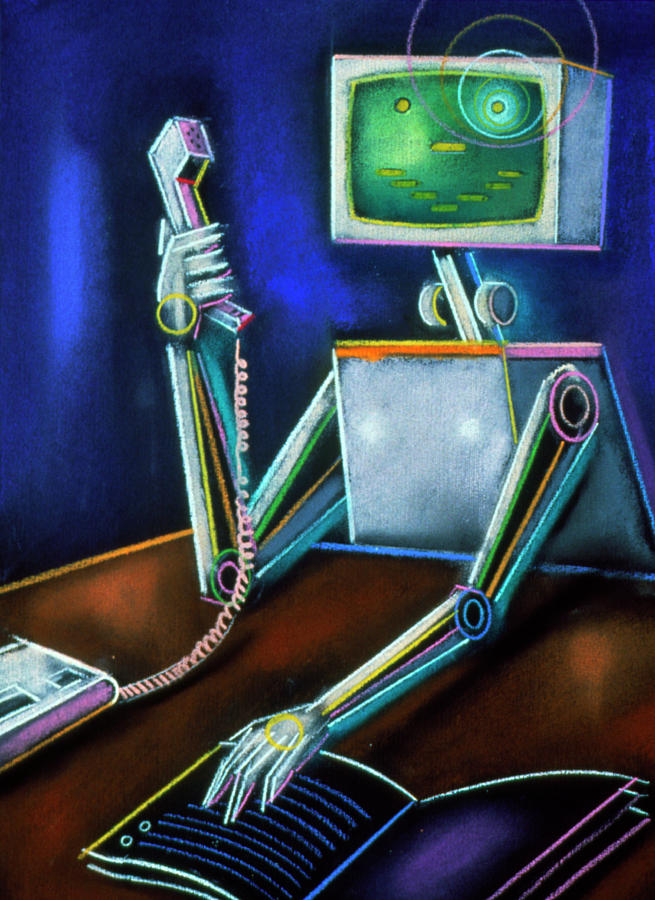In this pastel drawing, a somewhat abstract robot with a CRT-style monitor for a head stands prominently against a cloudy blue-black background. The robot's boxy head features a green screen displaying a crude, digital smiley face with hypnotic, multicolored rings radiating from the right eye. Its metallic body is adorned with vibrant neon highlights in blues, greens, pinks, and oranges. The robot’s right hand holds the handset of an old-style corded telephone, while its left hand rests on an open notebook placed on a brownish-orange desk. The detailed composition creates a nostalgic and intriguing scene, blending retro technology with a futuristic character design.